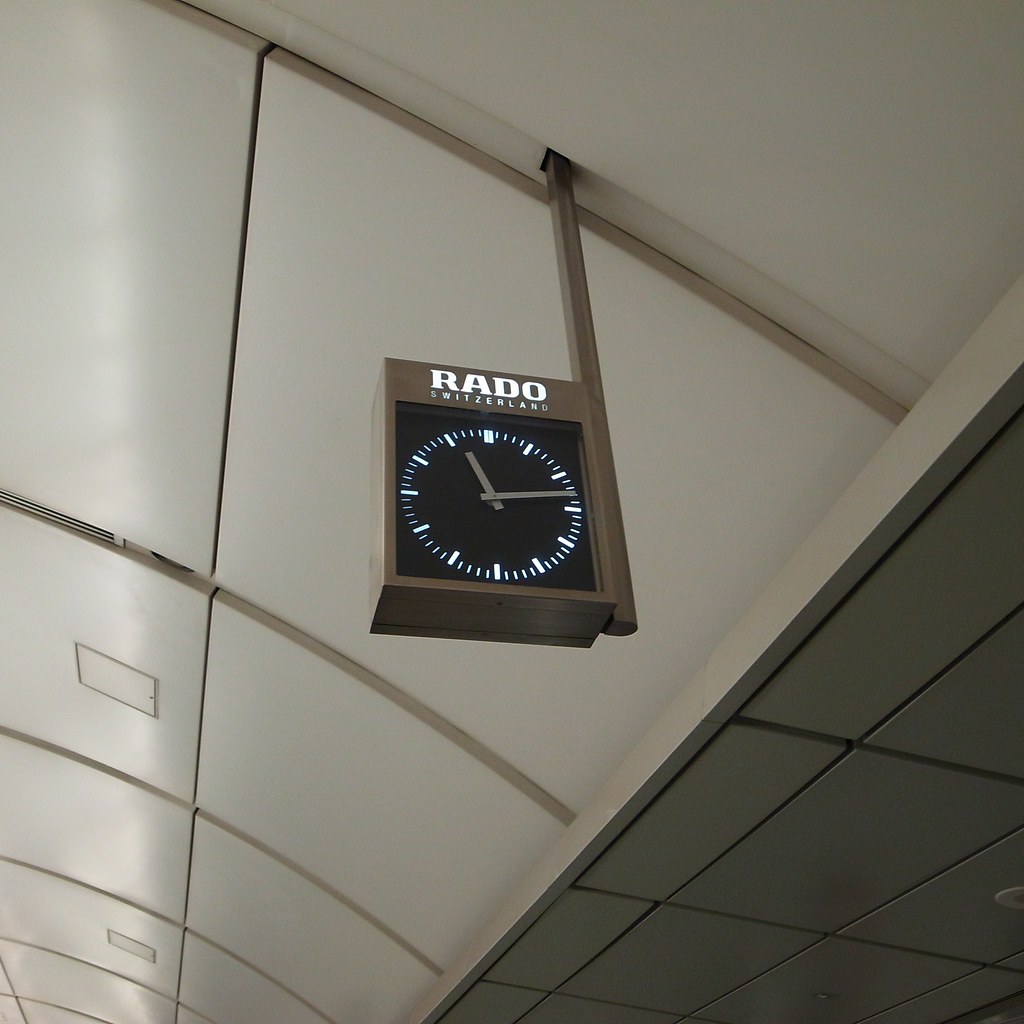This image features a Rado Switzerland-branded clock, prominently displayed in what appears to be a train station. The clock's design is reminiscent of nutritional facts labels, adding a unique and intriguing visual motif to its otherwise classic appearance. The current time displayed on the clock is 11:14. The background suggests a bustling public space, likely the inside of a modern train station, emphasizing both the utility and stylish design of the Rado clock. The clock's face is clear and easy to read, serving as a practical yet sophisticated timekeeping solution in a busy transit hub.